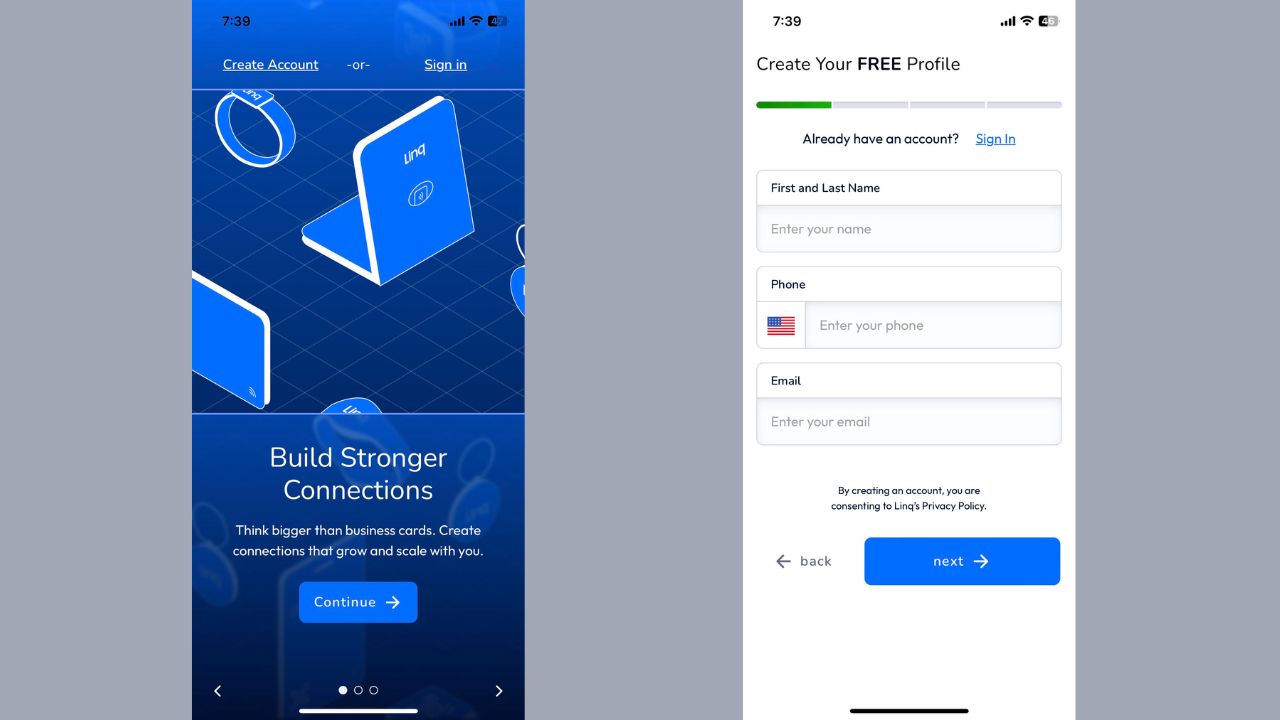This image consists of two mobile screenshots displayed side by side, creating a composite view of an app's user interface. On the left side, the initial screenshot shows a welcoming message encouraging users to create an account or sign in. The text promotes building stronger connections and thinking beyond traditional business cards, emphasizing scalable relationships. Below this message, there's a prominent blue "Continue" button with an arrow. The entire image is themed in blue and features various digital graphics, including a laptop, a smartwatch, and a tablet.

The right-side screenshot appears to be the subsequent screen, likely displayed after pressing the "Continue" button. This screen prompts users to create a free profile. At the top, there's a progress bar divided into four sections, with the first section colored green, indicating the user's progression through the setup steps. Below the progress bar, there's an option for users who already have an account to sign in, with the 'Sign In' text highlighted in blue. The form then requests the user's first and last name, phone number, and email address. At the bottom, there are "Back" and "Next" buttons for navigation, along with a disclaimer stating that by creating an account, the user consents to Ling's privacy policy.